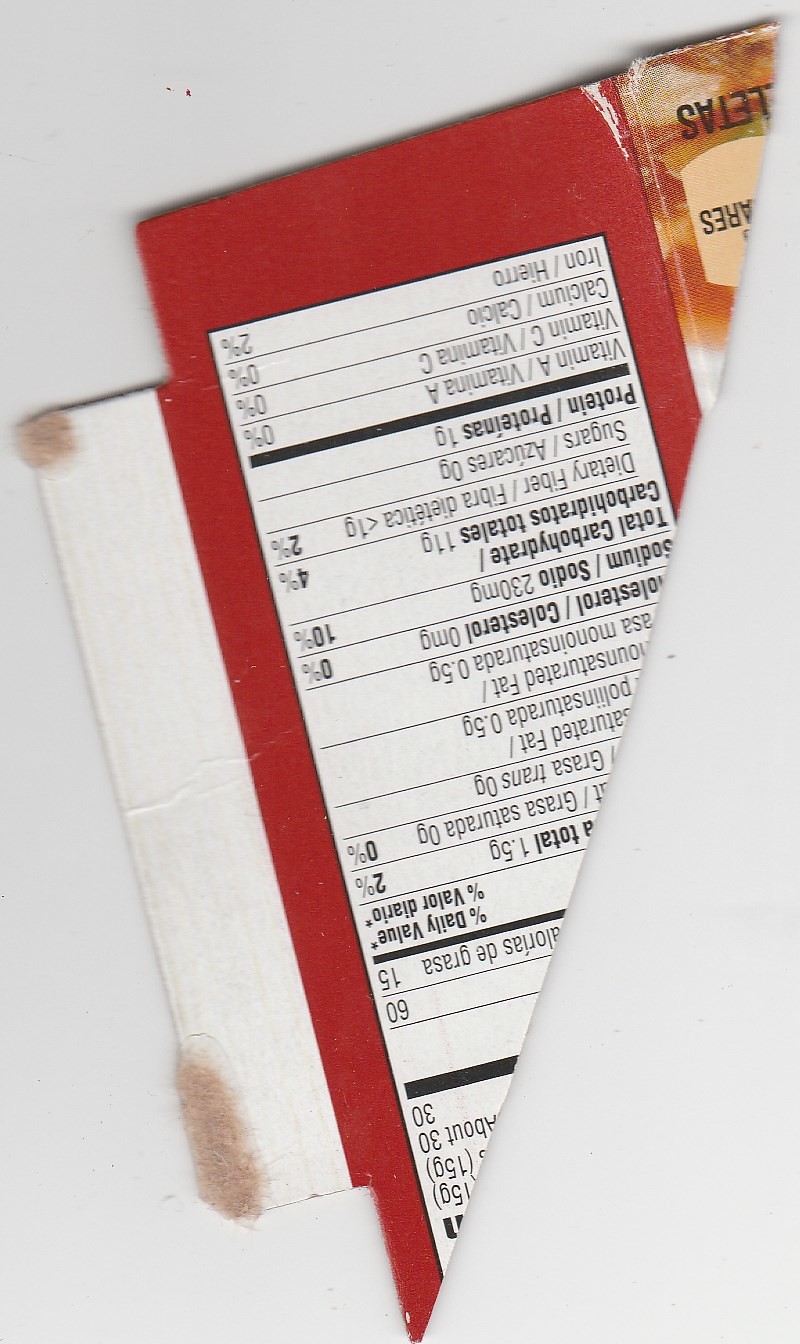This color photograph captures a complex composition involving multiple layers and cutouts. The primary focus is an upside-down segment of a food label set against a grey background. This image is positioned over another grey background, creating a layered effect that extends from the upper right corner to the bottom middle right. To further complicate the scene, a grey triangular shape intersects this area, suggesting the left side is part of another photograph that has been superimposed and trimmed to fit.

On the left side of the image, a smaller, diagonal, whitish card with brown markings at the top and bottom edges is visible. Adjacent to this is a reddish card featuring partially visible, black text of a nutritional food label, now rendered upside down. The legibility of the text is compromised due to the orientation and cropping. In the upper right section of the reddish card lies the diagonally cut portion of what appears to be a jar, displaying black text against its surface. This jar is bisected almost halfway, making it appear as though it represents part of the food product discussed in the label.